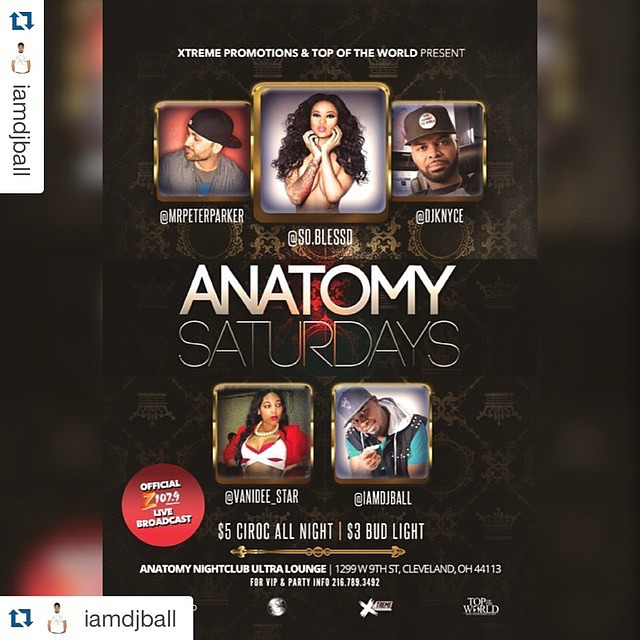The image is a detailed promotional flyer for Anatomy Nightclub and Ultra Lounge, located at 1299 West 9th Street, Cleveland, Ohio, 44113. At the top of the flyer, "Extreme Promotions and Top of the World Present" is prominently displayed. Below this header, there are three vertical images featuring headshots: a man on the left labeled @Mr. Peter Parker, a woman in the middle labeled @so.blessed, and another man on the right labeled @DJKNice.

The central portion of the flyer highlights "Anatomy Saturdays" flanked by two more images: a woman on the left labeled @thevanity_star and a man on the right labeled @IAmDJBall. 

The flyer details the event offerings including $5 Ciroc all night, $3 Bud Light, and mentions an official 107.9 live broadcast. At the bottom, VIP and party information can be obtained by calling 216-789-3492.